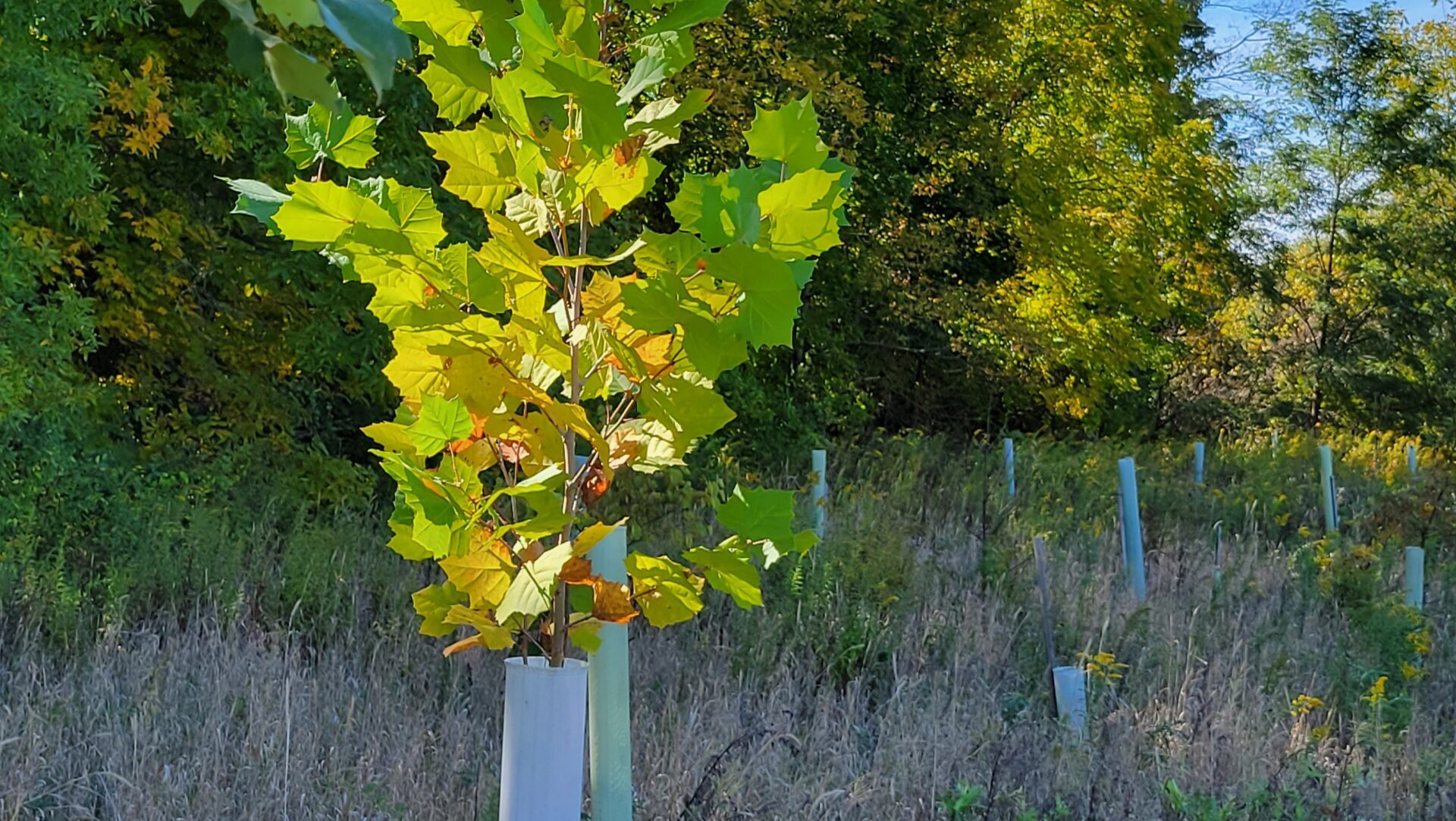On a bright, sunny day, the image captures a densely packed area of a small forest or hill covered with tall, high-rising grass and weeds, giving a sense of natural wilderness. The sky peeks through the canopy, revealing hues of blue with scattered white clouds. The sunlight illuminates the scene, casting a natural glow on the lush greenery. In the foreground, a thin, young tree with a mixture of green and some yellow leaves emerges from a white tube and blue tube support, indicative of recent planting efforts. This young tree contrasts with the backdrop of mature, fully grown green trees, some showing hints of yellow and orange foliage. Scattered throughout the grassy area are multiple similar blue poles, which are supports for new trees. Among these, only one of the poles hosts a growing tree; the others await their turn. The very high grass, some of which appears dried out, surrounds these poles but stops before the tree line, creating a clear separation between the grassy area and the dense forest beyond.